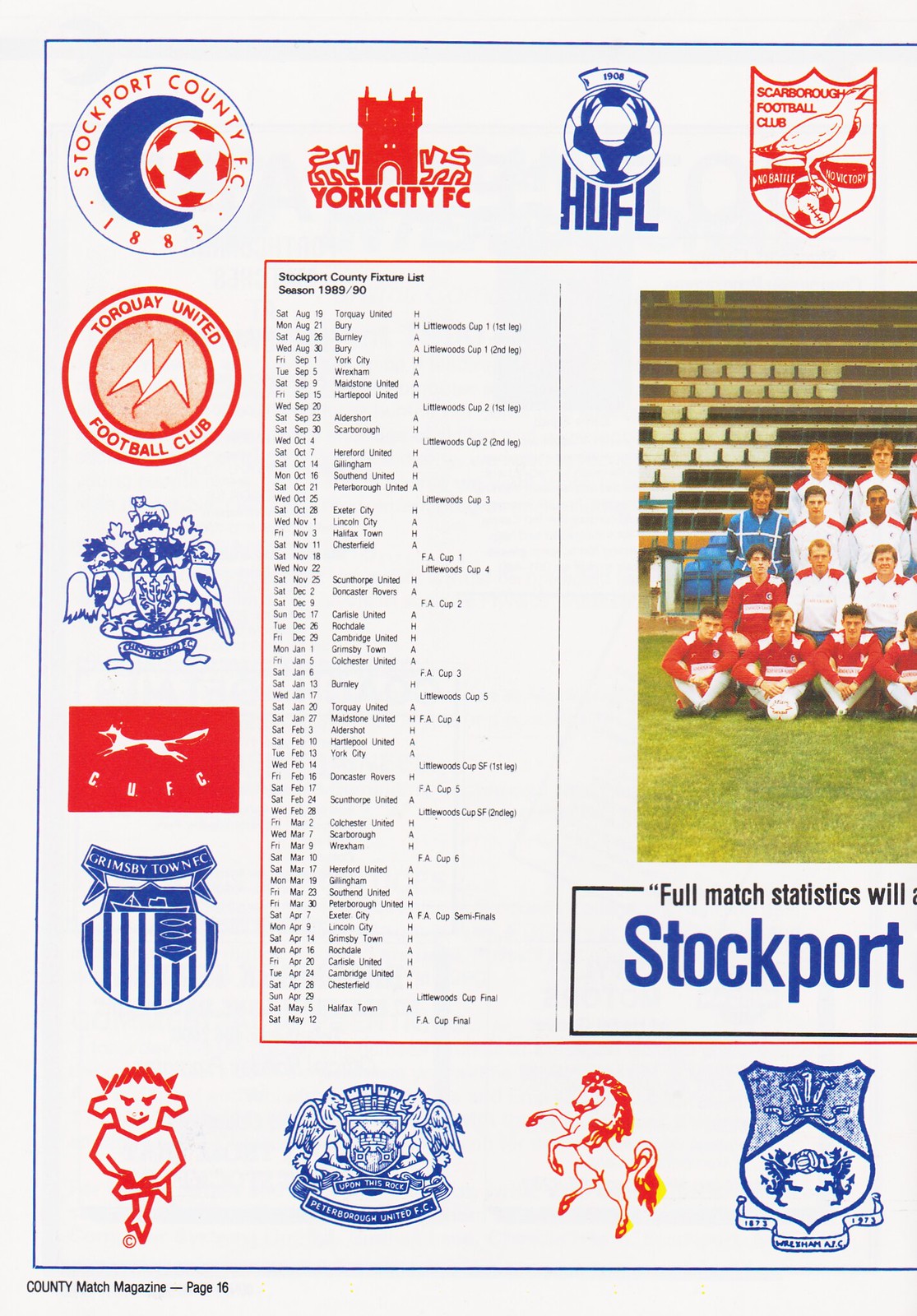The image is a partial photograph of the left half of a program page from a soccer game, primarily featuring Stockport's team. The background is white, adorned with various colorful logos and insignias from different football teams—some in red, some in blue, and some combining both colors. Along the top and down the left side, as well as across the bottom, are numerous team logos, including ones labeled York City and H-U-F-L, alongside a round logo and a shield with text. There's also an image resembling a devil at the bottom left.

In the center of the image, a red-outlined section features a sequence of dates likely representing a schedule, though the black print is too small to read. To the right of this section is a partially visible photograph of Stockport’s team posed on a field. The front row shows players in red, seated, with a couple of players in white kneeling behind them. Further back, two rows of standing players include more in white and one in blue, with stadium bleachers in the background.

Below the photograph, partially visible text reads: "full match statistics will," followed by the word "Stockport" in large blue letters, indicating the cut-off nature of the page.